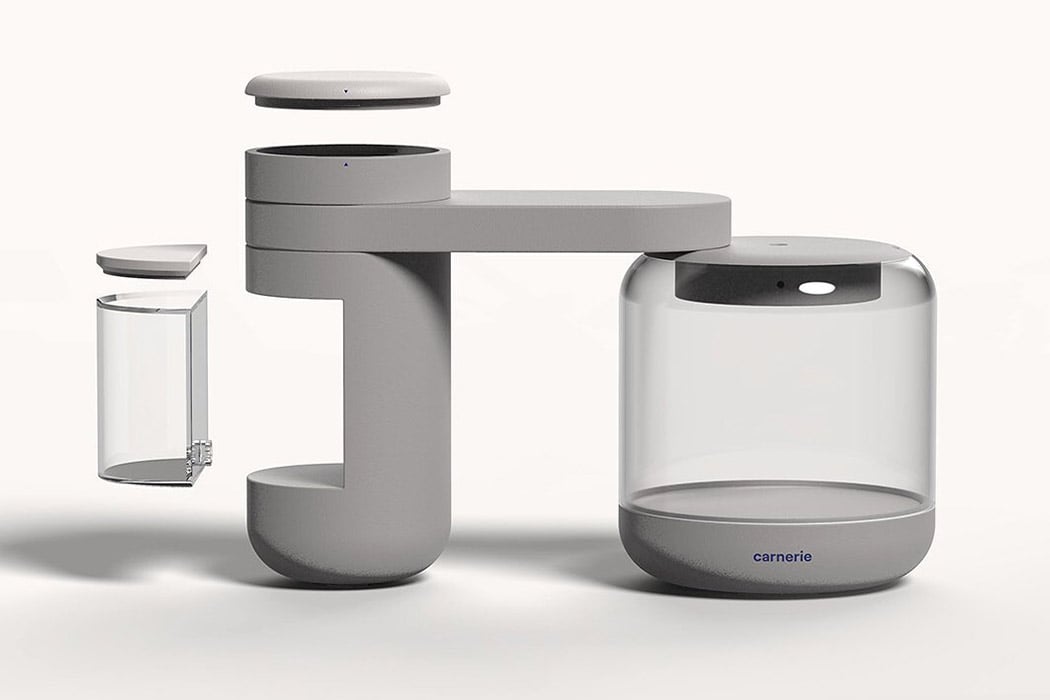This rectangular image, measuring approximately six inches wide by four inches high, features a kitchen appliance set against a background that transitions from a very pale pink at the top to a light gray in the center, and then to a darker gray with pink tones at the bottom corners. 

At the center of the image is a detailed view of the appliance's components. On the left side, there's a semi-circular glass container with a flat bottom and a cap on top. This glass container appears to be inserted into an indented section of a vertical cylinder made of light gray plastic. This vertical cylinder, which consists of four layers, has a rectangular cutout on its left-hand side and an extended arm at the top connecting it to the main part of the appliance.

The main cylindrical component on the right side of the image is wider and appears to be made of plastic with a clear central section and light gray top and bottom parts. This portion of the appliance is designed to lay underneath the extended arm, which links the left glass container to this central cylinder.

At the very bottom of the appliance, the brand name "Carnerie" is displayed in bold black print against the gray base of the glass. The setup suggests this appliance could possibly be a blender, a coffee maker, or a high-end kettle, although the exact function is indeterminate based on the visible components.